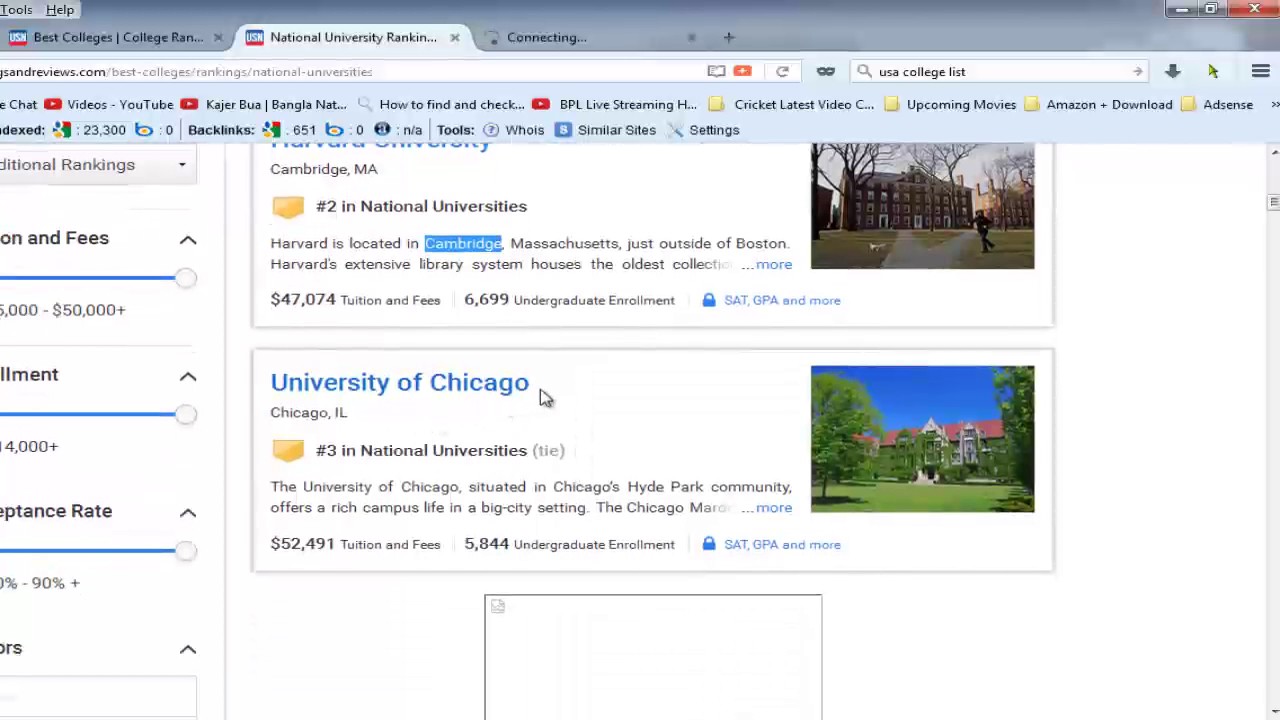The image depicts a webpage related to National University Rankings, as indicated by the browser tab. The top of the webpage appears cluttered with a light green and light blue bar spanning across the top, containing various links and icons. Some of the links include red icons indicative of YouTube, while others feature yellow icons.

In the main content area of the webpage, there is an incomplete list of universities ranked nationally. The top portion of the page is either cut off or scrolled up, hence the number one ranking is not visible. However, the page prominently displays Harvard University as the number two ranked national university. Accompanying this ranking is an image of one of Harvard's buildings, along with a brief description noting its location in Cambridge, Massachusetts, just outside of Boston. It also mentions Harvard's extensive library system, which houses the oldest collection.

Below this, the University of Chicago is listed as number three in the national rankings, featuring an image of one of its buildings surrounded by lush greenery. There is an empty space under the University of Chicago entry, indicating either a missing image or content that hasn't loaded.